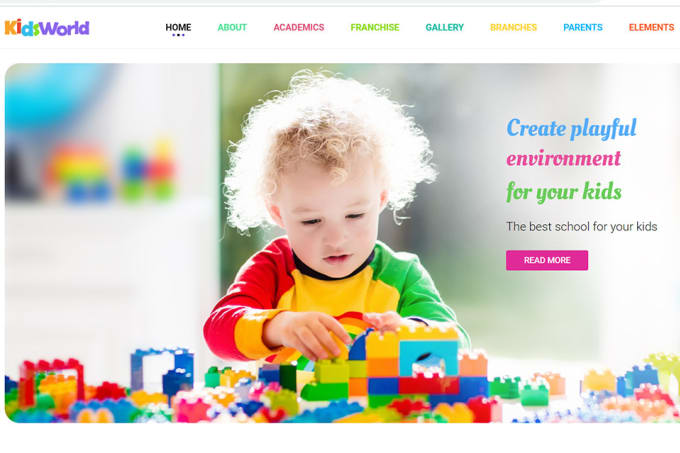The landing page of the Kids World website features a vibrant and engaging layout, designed to catch the eye of both children and parents. Across the top, a colorful navigation menu includes links for "Home," "About," "Academics," "Franchise," "Gallery," "Branches," "Parents," and "Elements." The "Home" tab is in plain black, while the other tabs are displayed in various bright colors, creating a rainbow effect.

Below the navigation bar, a heartwarming image depicts a curly-haired child wearing a multicolored shirt with a red sleeve, green sleeve, yellow body, and black collar. The child is deeply engrossed in playing with Duplos, which are scattered on the floor and match the vibrant colors of the navigation tabs above.

To the right of the image, a cheerful message is displayed in playful fonts. It begins with "Create Playful" in light blue, followed by "Environment" in a light purple shade, and concludes with "for your kids" in bright green. Below this message, a bold statement reads, "The Best School for Your Kids," accompanied by a clickable button for more information, which is also in a bright color.

This lively and detailed design gives a joyful and inviting impression, perfectly capturing the essence of an engaging and nurturing environment for children.